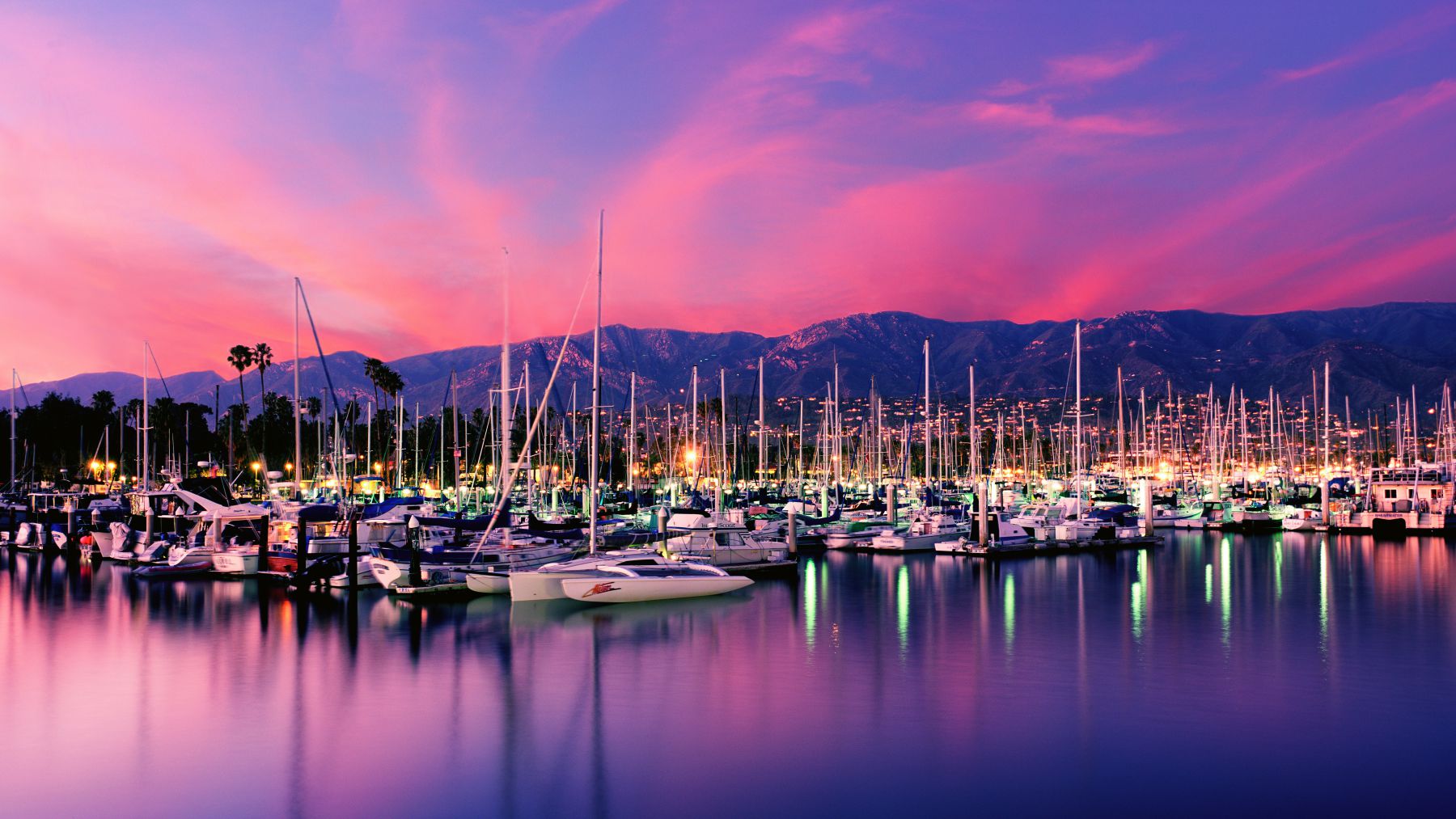The photograph captures a serene marina at dusk, where numerous small sailboats are moored along multiple docks, creating a forest of vertical masts that rise into the tranquil evening air. The sun has already set behind a distant mountain ridge, casting a stunning array of purples, pinks, and blues across the sky. These vibrant hues of the twilight sky are mirrored in the calm waters of the harbor, intermingling with the reflections of the sailboats' masts and a few scattered streetlights on the docks. To the left, there are palm trees and other foliage framing the scene, while to the right, faint, low-lying city lights glimmer at the foot of the mountains. The boats, mostly white with their sails down, add to the peaceful and calming ambiance of this picturesque moment, devoid of human activity, emphasizing the stillness and beauty of the scene.